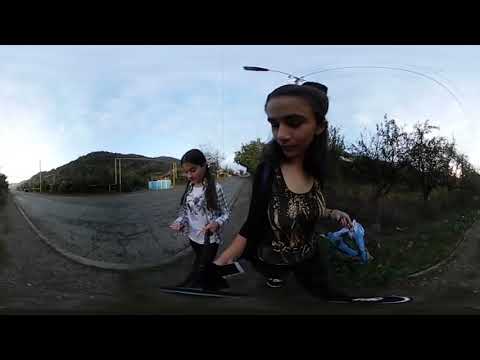This image is an outdoor, daylight selfie of two young women, characterized by a curved and distorted visual effect typical of a 360-degree or panoramic camera lens, creating a stretched and rounded appearance. Both have long, dark brown to nearly black hair. The woman on the left wears her hair in two pigtails and is dressed in a long-sleeve white shirt with black and gray designs, black pants, and black shoes. The woman on the right has her hair pulled back and is dressed in a black blouse adorned with white and tan designs, black pants, and a black cardigan. She clutches a phone in her right hand and something blue is either in her hand or on the ground behind her.

The scene's background includes a road to the left, which is asphalted but cracked and currently void of any vehicles. There is a streetlight directly behind the women, extending over the road. The backdrop also features small bushes, green trees, and a distant tall hill covered in lush greenery. Above them, the sky is a light blue, dotted with white clouds, lending a calm atmosphere to the image. Black bars on the top and bottom of the frame give the impression that this is a still image captured from a video.